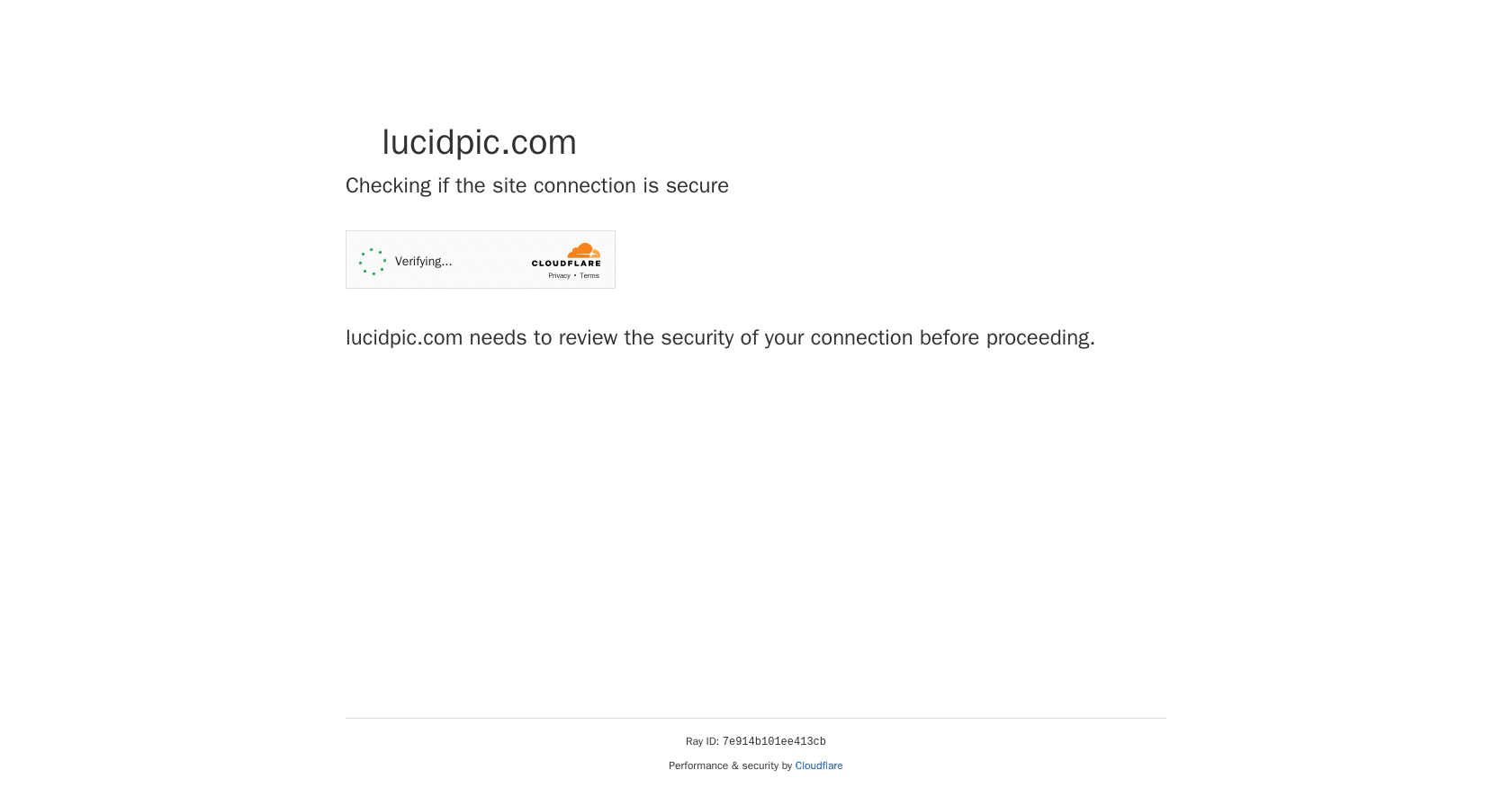This detailed caption describes a security check page from CloudFlare:

"This is an image of a security verification page encountered on the website lucidpick.com, implemented through CloudFlare's security services. At the top of the page, the domain name 'lucidpick.com' is prominently displayed. Below it, a message indicates that the site is in the process of establishing a secure connection. Another message reads 'Verifying...' accompanied by a rotating circle, signifying that the system is currently validating if the user is human or a bot. There is a small CloudFlare logo next to the text 'Privacy & Terms,' which likely links to CloudFlare's privacy policy. At the bottom, a unique identifier called a 'Ray ID' is shown, serving as a specific CloudFlare network identifier for this security check."